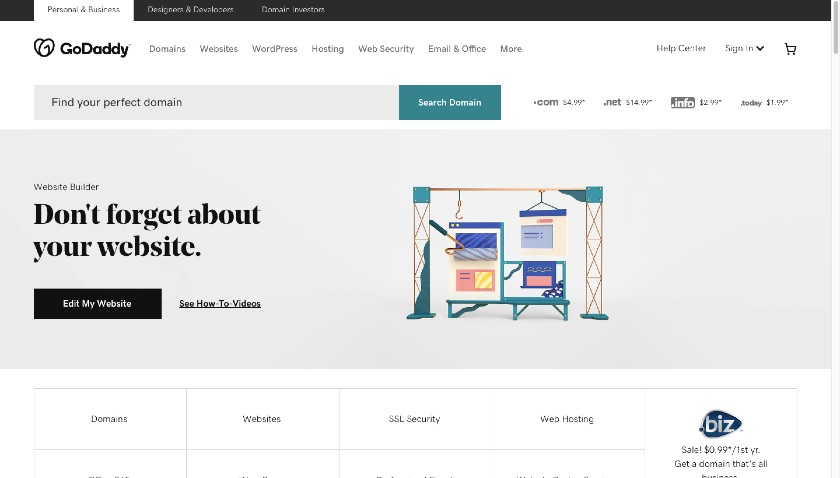This image is a detailed screenshot from a GoDaddy website, presumably viewed on either a desktop PC or a laptop. The format is a long rectangular shape, wider than it is tall, characteristic of a typical browser window. The screenshot exhibits a white background, accented by the GoDaddy branding prominently displayed in the upper left corner.

The GoDaddy logo, which features a simplistic, almost heart-like black symbol composed of a single swirling line, is immediately noticeable. Adjacent to the logo, the name "GoDaddy" is presented in a single word with black text. To the right of the logo are several clickable links leading to different sections of the website, including "Domains," "Websites," "WordPress," "Hosting," "Web Security," "Email & Office," and a "More" option indicating additional categories.

Further right on the navigation bar, there are links to the "Help Center," a "Sign In" button with a drop-down arrow for additional options, and a shopping cart icon for easy access to purchases. Below this primary navigation bar lies a prominent search bar with the placeholder text "Search Your Domain" and a green button for executing searches.

Beneath the search bar, there is a significant visual element—a large clickable advertisement or link with the text "Edit My Website." This link likely directs users to their website dashboard or login page. The visual accompanying the link is a creative illustration of a machine assembly line, metaphorically representing the process of creating different websites with a variety of physical devices.